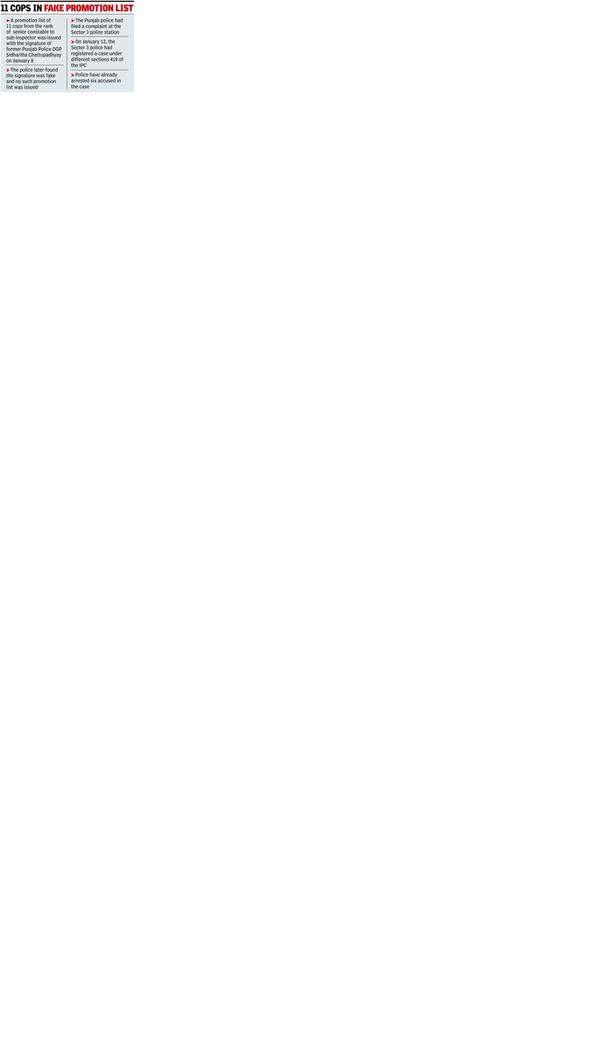The image is a diminutive screenshot or photograph capturing an informational page. At the apex of the image, the title prominently reads "11 Cops in Fake Promotion List." The words "11 Cops in" are emboldened and displayed in black, while the remaining portion of the title, "Fake Promotion List," is equally bold but rendered in a red-orange hue. Unfortunately, the actual paragraphs or detailed content beneath the title are indiscernible due to the image's minuscule size. The subsequent text below the headline is printed in black, though its specifics remain elusive.